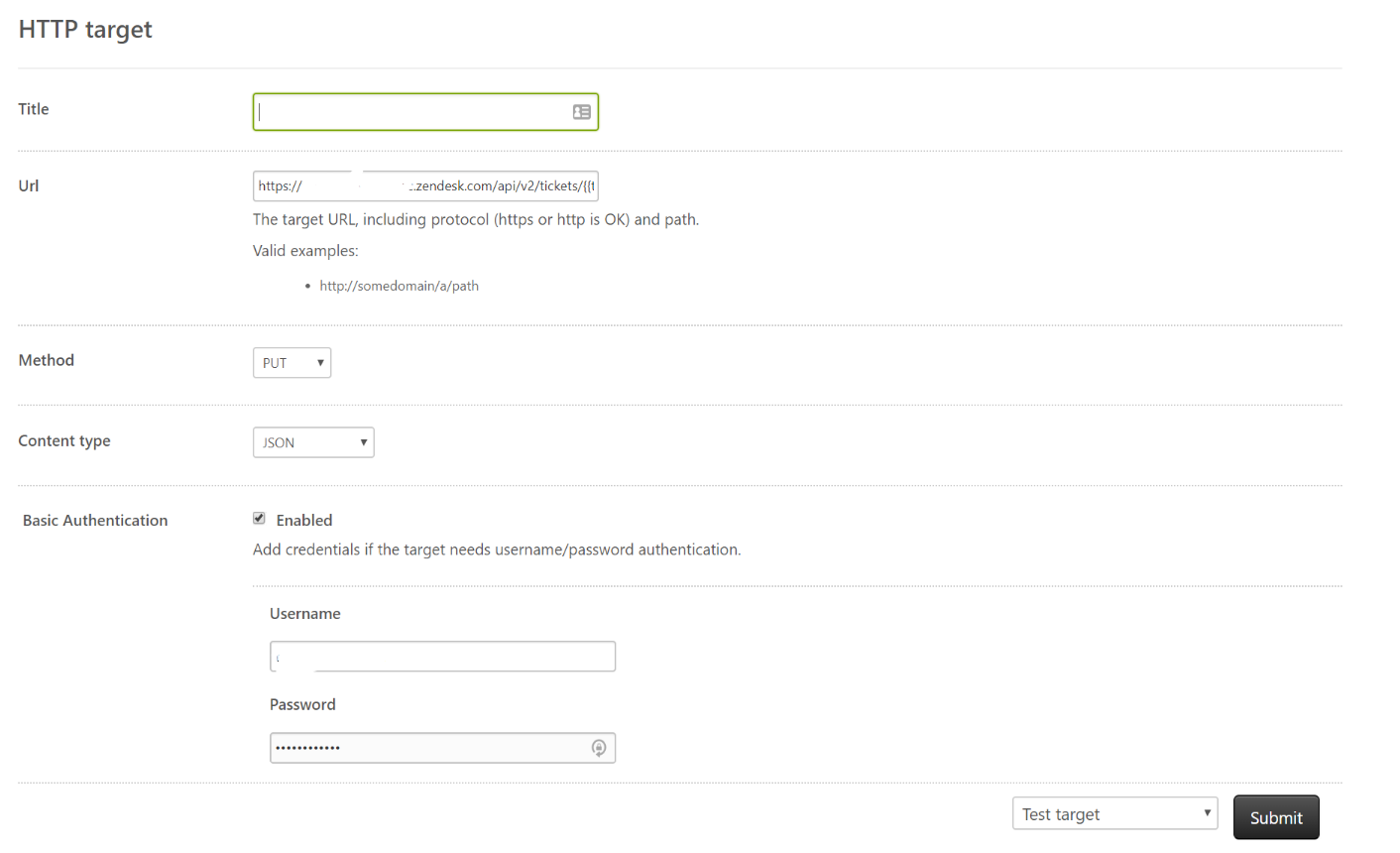The image depicts a web configuration interface with several sections outlined as follows:

- **Top Left:** A section labeled "HTTP Target" in black text.
- **Title Section:** Contains a text input field edged with a green rectangular border.
- **URL Section:** An input field for entering a URL, along with a description below it that reads, "The target URL, including protocol (HTTPS or HTTP), is okay. Path and valid examples are provided below." An example URL is presumably shown beneath this description.
- **Method Field:** Currently set to "PUT."
- **Content Type:** Set to "JSON."
- **Basic Authentication:** This section is marked as "Enabled" with a checkmark. An option to "Add credentials if the target needs username/password authentication" is present.
- **Credentials Fields:** Two input fields, one for "Username" (currently empty) and one for "Password" (with ten dots indicating a hidden password). Both fields are labeled in black text.
- **Background:** The entire interface is set against a white background.
- **Bottom Right:** A "Test Target" button accompanied by a black "Submit" button to its right.

This detailed interface is designed for configuring and testing HTTP targets, incorporating input fields and options for method selection, content type, and authentication.